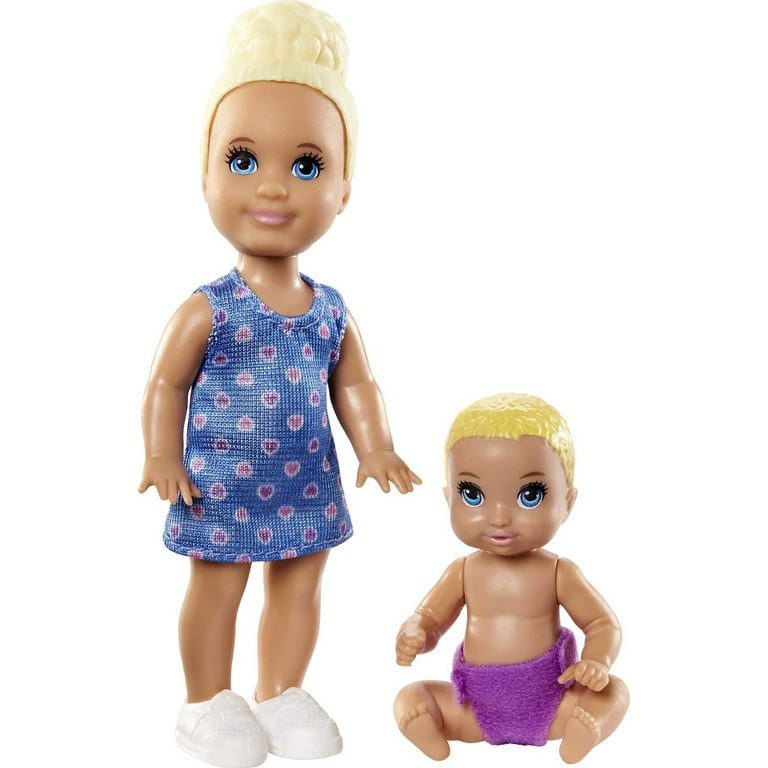This photograph displays two caramel-colored dolls with bright turquoise blue eyes and blonde hair. The doll on the left portrays a young girl and is dressed in a blue sleeveless dress adorned with small, purple hearts and red berry-like decorations. She wears white shoes and a yellow knit hat, with her hair tied up in a bun. This taller doll, about twice the height of the infant, has her arms down at her sides with fingers fully extended and pink lips. The doll on the right is a baby, seated and wearing a purple diaper that resembles shorts. The infant doll has balled-up fists, yellow hair, and similar blue eyes and pink lips.